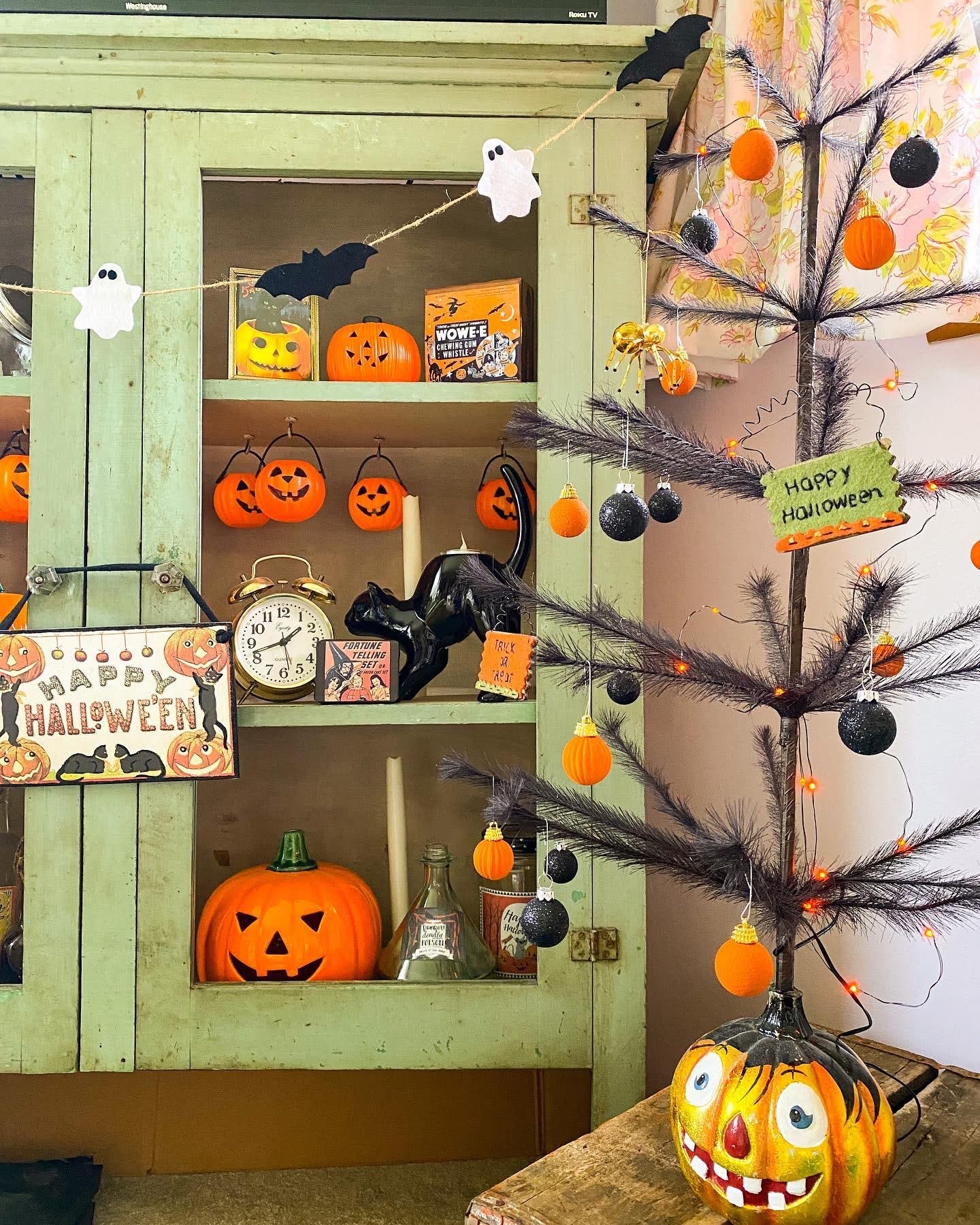This photograph showcases an elaborate Halloween display centered around a vintage, wood-framed Curio cabinet, painted in a faded grassy green hue. The cabinet's open front reveals three shelves filled with a delightful assortment of spooky decorations. Among them are multiple small plastic pumpkins, a larger ceramic pumpkin, an antique-style alarm clock, and glass bottles. A notable piece is the black cat statue designed to hold a candle on its back. Enhancing the eerie ambiance, a festive sign reading "Happy Halloween" hangs from the cabinet's door handles. Draped across the top of the cabinet is a string adorned with black bat and white ghost cutouts, each ghost featuring stark black eye sockets. 

To the right of the cabinet stands a Halloween-themed pine tree, reminiscent of a scrawny Christmas tree but painted black. This tree is festooned with shiny black and orange pumpkin-style decorations, orange fairy lights, and small spiders, adding a creepy charm. The tree is also adorned with a small sign proclaiming "Happy Halloween" and is rooted in a ceramic pumpkin base with a clown face, resting atop a table. The scene evocatively captures the essence of Halloween with meticulous attention to festive, spooky details.